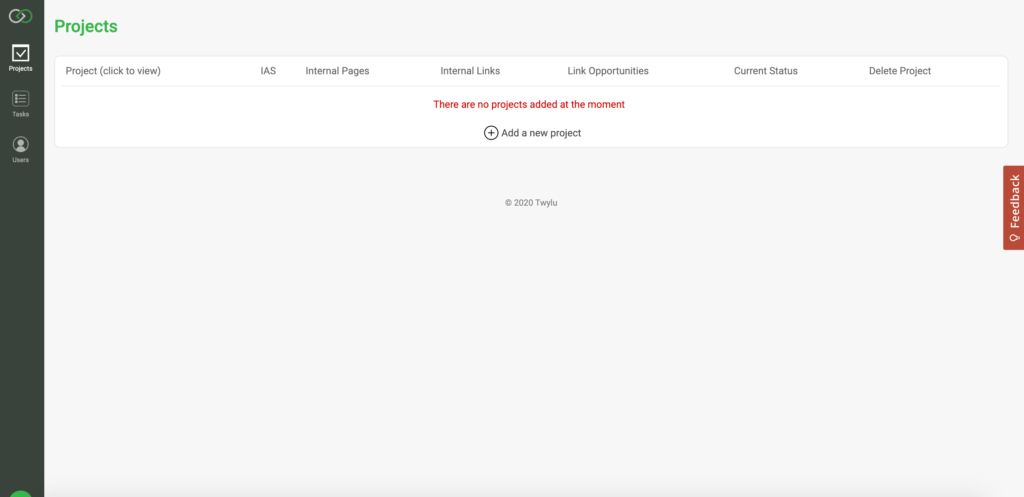In the upper left-hand corner of the image, there's a vertical black bar with two overlapping circles at the top—one white and the other green. Below these circles, the bar features three icons labeled "Projects," "Tasks," and "Users," respectively. To the right of this menu bar lies the main window of the page. Currently, there are no projects added, so the window displays six placeholder titles: "Project," "Click to View," "IAS," "Internal Pages," "Internal Links," "Link Opportunities," "Current Status," and "Delete Project." Additionally, an "Add New Project" button is visible, prompting users to initiate a new project.